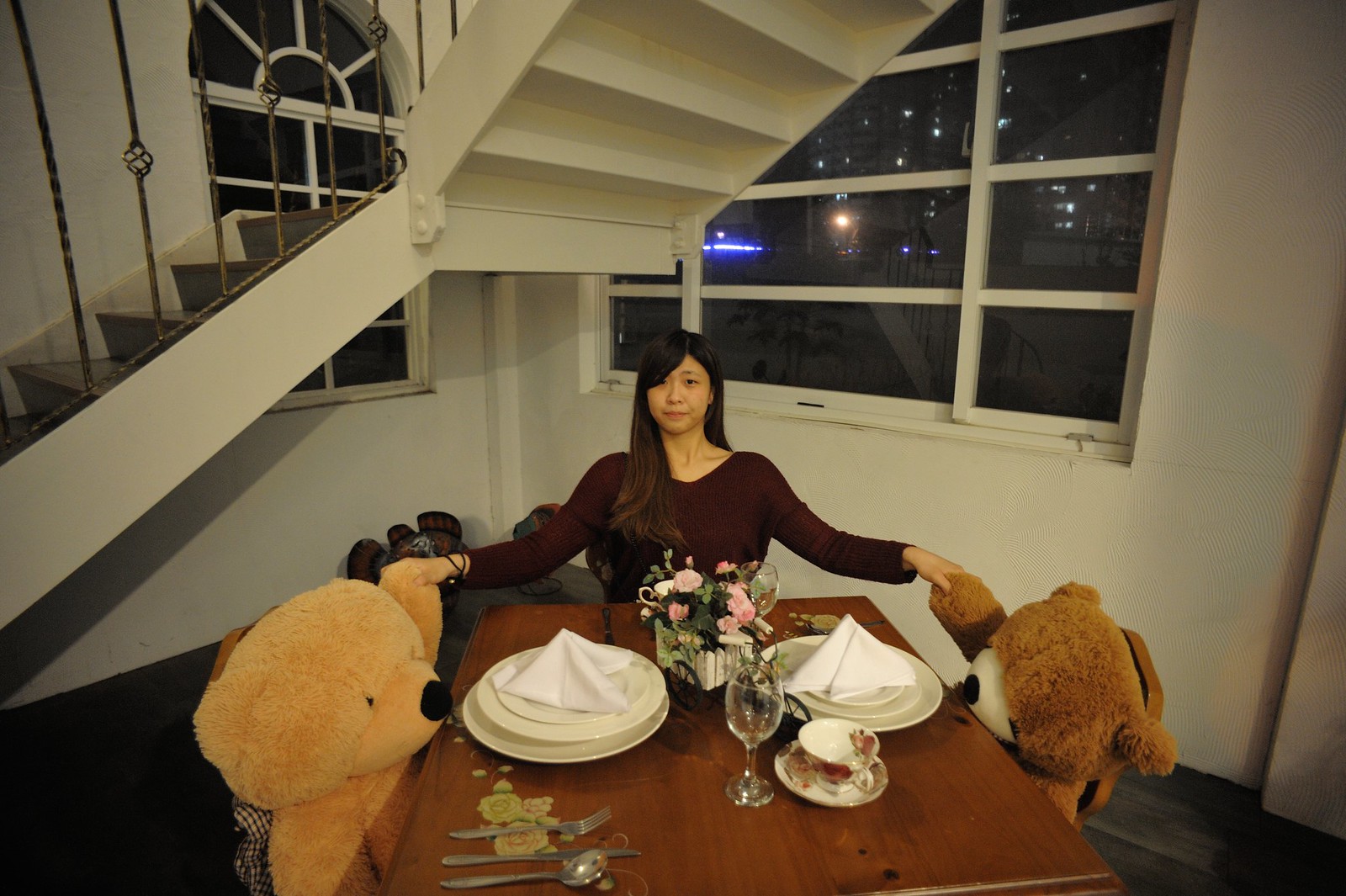In this color indoor photograph, a young Asian woman with long dark hair, dressed in a maroon long-sleeved sweater, is sitting at a brown dining table set beneath metal stairs that ascend from the left and reach the middle top of the image. Behind the stairs are large windows revealing a nighttime cityscape with illuminated buildings. The table is adorned with a white tablecloth, folded napkins atop stacked plates, and a vase of pink flowers arranged in a white picket fence-style square container. Clear glass wine glasses, teacups with brown patterns, and silverware complement the place settings. The woman is flanked by two large child-sized teddy bears—one tan on her left and the other darker brown on her right—and holds hands with both of them. She gazes directly at the camera, framed by this whimsical and warmly-lit indoor scene.